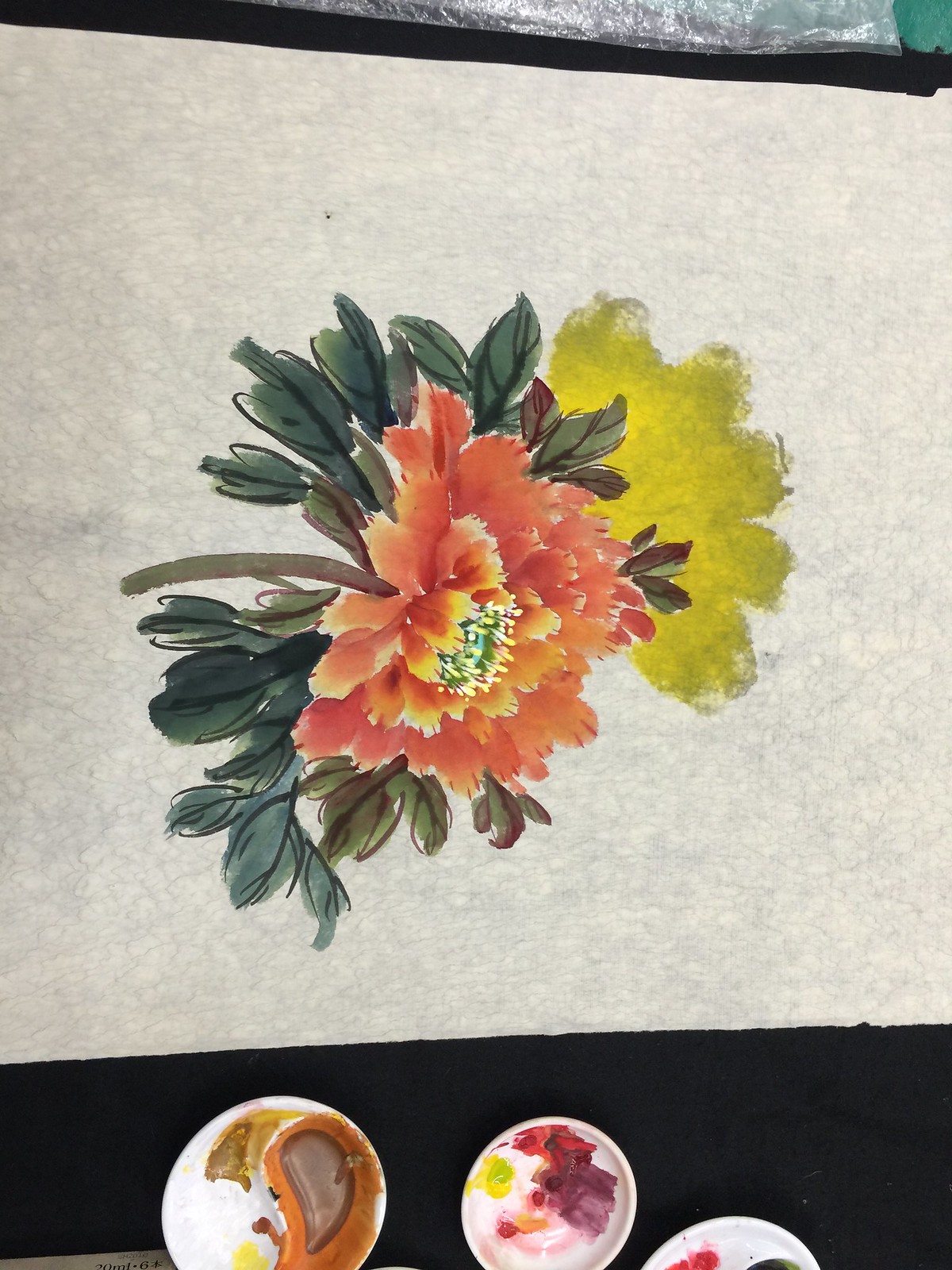This image showcases a watercolor painting on a white piece of paper, which has been turned sideways. The composition features two distinct flowers. The first flower, positioned on the right, is entirely yellow and appears plain. Below it, the second flower stands out with its vivid reddish-orange petals accented by yellow and orange highlights, and a green center. Green leaves encircle this flower, extending from its base to its top, accompanied by a green stem protruding downward.

In the painting’s background, a black board or palette supports the white paper, within which the artwork is stretched. At the bottom of the image, there are three round tubs of paint. The leftmost tub contains a mix of brown, white, and a little yellow. The middle tub shows a blend of purple, red, yellow, and white, while the rightmost tub contains traces of purple. Scatterings of silver and green are also visible in the background, hinting at the surrounding environment.